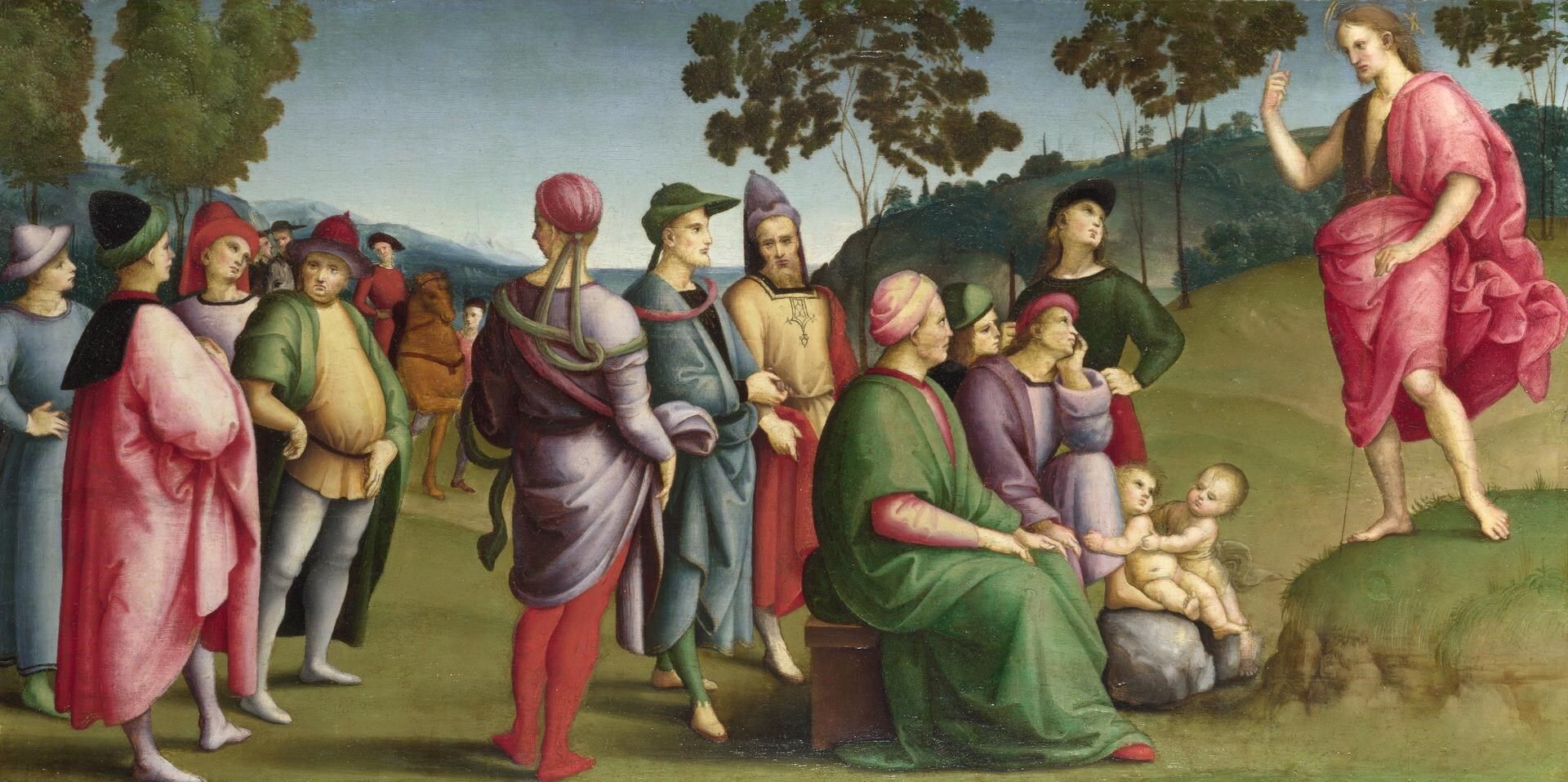In this renaissance-style painting, likely hailing from the 1500s or 16th century, a central figure who could be Jesus stands on a grassy mound. He is draped in a reddish-pink robe with a darker garment underneath, his skin mostly bare, and he has light brown, long hair. With one hand raised, he appears to be addressing a crowd. Surrounding him are about 12 to 15 people, including a couple of small children near his feet, clinging to another seated figure. The attendees are dressed in colorful robes and cloaks characteristic of the era. The setting features a vibrant green meadow with rolling hills and scattered trees in the background. The sky transitions from blue to a brighter hue nearer to the horizon. Additionally, a man on horseback is visible, adding to the scene's dynamic composition.